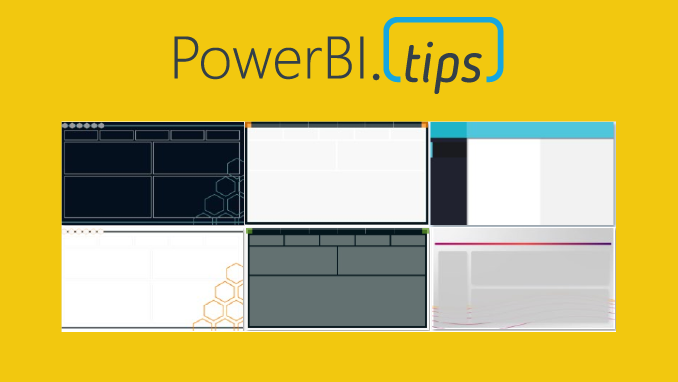The image is a screenshot showcasing a brand or product logo for "PowerBI.tips," with the main text written in a bold, italic sans-serif font. The text "PowerBI" is followed by ".tips," with the ".tips" enclosed in a blue, curved rectangular outline that breaks around the word. The background is a vivid yellow rectangle that contrasts with the blue outline around "tips."

Beneath the text, there are six rectangular grid sections arranged in two rows of three. These sections are blank and resemble computer screenshots or website templates. The templates are displayed in various black and white grids, some with accents of other colors. The top left template has a honeycomb pattern with a black background outlined in grey. The top middle features black outlined rectangles with grey interiors. The top right contains a mixture of black, white, and grey boxes with a blue rectangle overlay. For the bottom row, the leftmost template repeats the honeycomb pattern but with a white background and gold outline. The middle bottom template showcases another design theme in white and grey. The bottom right template is lighter grey with a touch of red and purple lines in it. Overall, the designs appear to be basic wireframes or placeholders, as they lack specific text, icons, or buttons.